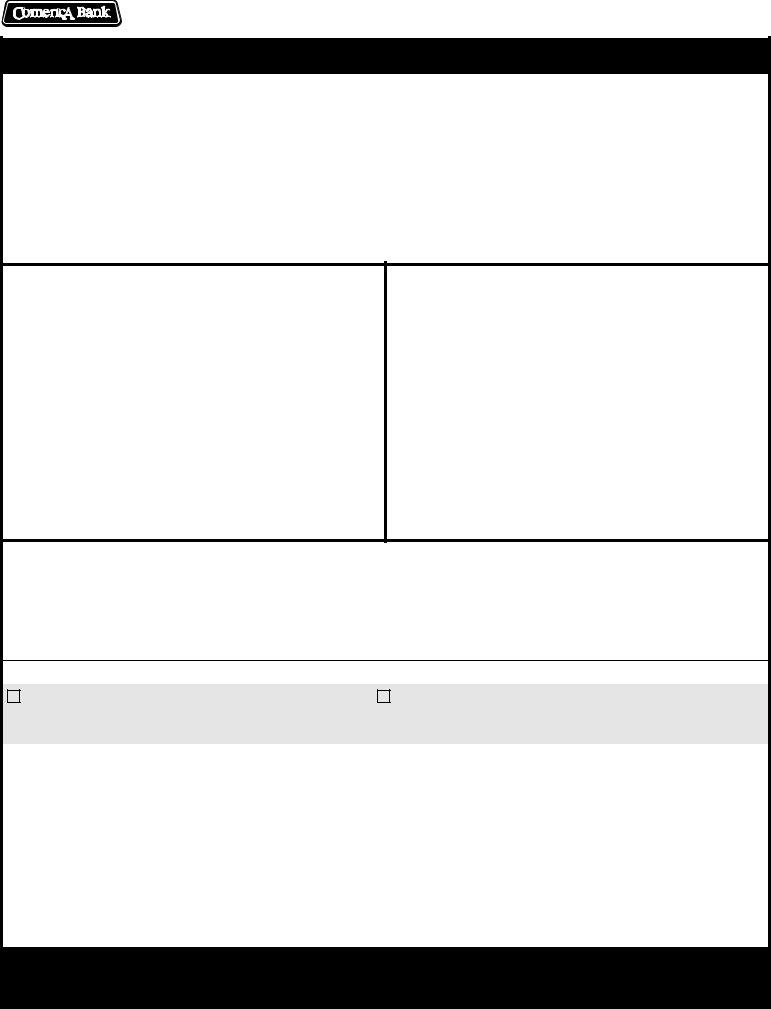The image depicts a blank website layout, structured in a detailed manner. At the top left, there's a badge in black featuring white lettering that appears to read "Comerica Bank." Below this, a black panel approximately a centimeter thick spans the entire width of the screen. Directly underneath, there's a large white rectangle, currently empty. Beneath this white section, the space is divided into two separate rectangles, each shorter in length but taller in width compared to the area above. Below these sections, there's another rectangle that spans the full width of the screen and is narrower than the topmost black panel. A very fine grey line lies beneath this section, followed by a narrow white panel about half a centimeter thick, also extending the full width of the screen. Subsequent to this is a grey panel running across the screen's width and measuring about one and a half centimeters in height; within this grey area sit two small white squares, positioned in the far left corner and center, respectively. The next segment is a white panel approximately three centimeters high, covering the entire width of the screen. Finally, at the bottom of the layout, there's a black panel around a centimeter high, stretching across the screen's complete width.